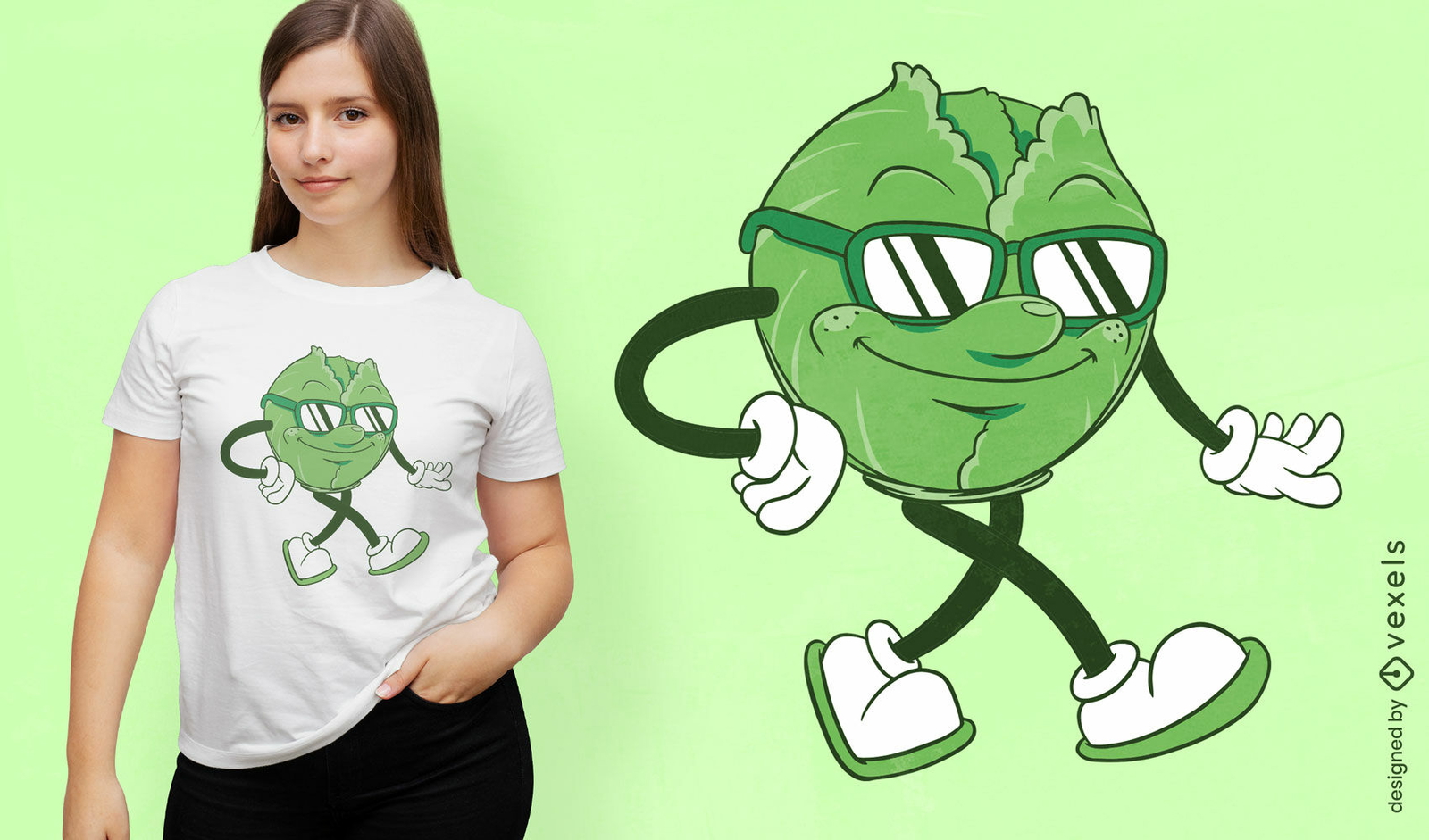The image features a young woman with long reddish-brown hair and fair skin, wearing a white crewneck t-shirt and black jeans. Her left hand is tucked into her jeans pocket while her right arm hangs by her side. The white t-shirt displays a whimsical cartoon graphic of a green cabbage head character. The cabbage head sports playful green sunglasses with black-striped lenses, a bulbous nose, and a friendly smile. Completing the look, the cabbage has black, stick-like arms and legs, white gloves with puffs around the wrists, and white shoes with green soles. The background of the image is a light mint green. On the right side of the image, there is a detailed close-up of the cartoon cabbage graphic, highlighting the same distinguishing features. The overall scene gives an impression of an advertisement for t-shirts with unique, playful designs.